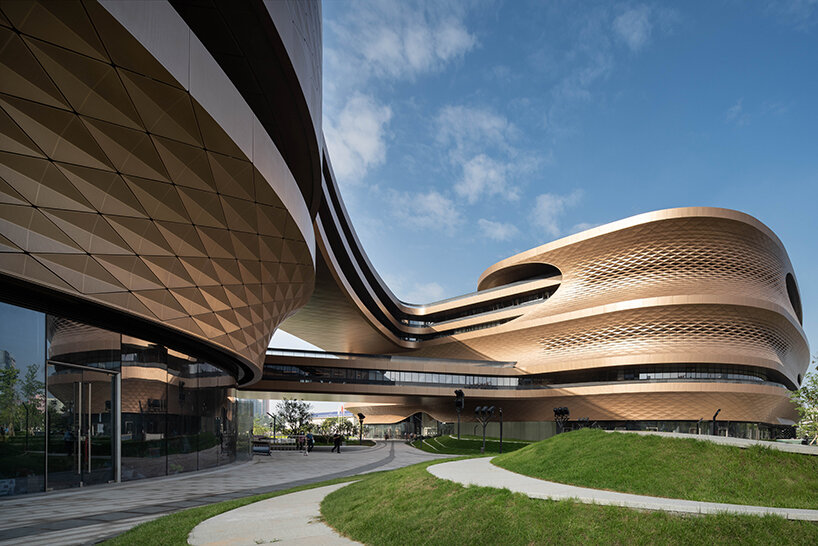In the image, there is a very modern and architecturally striking building featuring smooth, rounded curves on the outside, enveloped in gold or copper triangular plates that form an intricate, cross-hatched design. The structure consists of two large, rounded components connected by two distinctive skywalks; a larger, two-story upper skywalk with windows, and a smaller lower hallway. Beneath these connecting sections, a glass-walled ground floor with diamond-patterned doors and extensive windows wraps around both structures, providing clear visibility into the interior. In the foreground, there is a spiraling grass area situated towards the front and left side of the image, while further left, a sidewalk or road is evident. There are small figures of people walking, indicating the scale of the structure. Scattered trees, street lights, and other modern buildings are visible in the background, contributing to the overall scene.